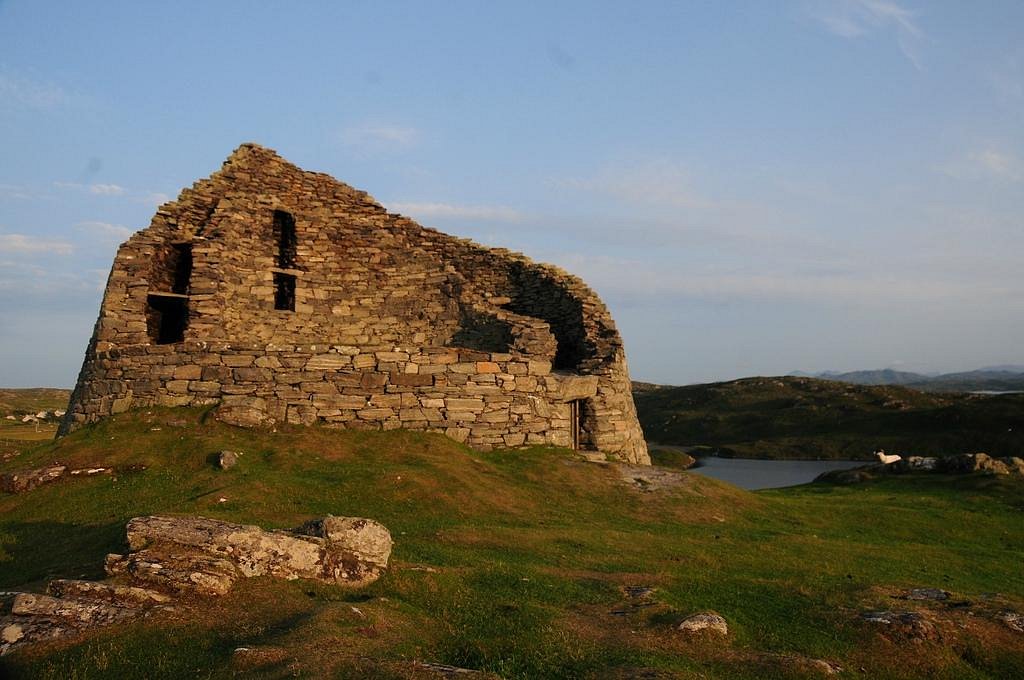The image depicts a color photograph of an old, crumbling stone structure that appears to be the ruins of a house or part of a castle. The dilapidated building is constructed of layered stones and features stone steps in the forefront left lower corner. Much of the structure is missing, revealing its interior and several broken windows. A door is noticeable on the lower right side of the structure. Surrounding this ruin are lush green hills, dotted with a considerable number of sheep, stretching out into a background that includes a body of water, possibly a river or pond. Further in the backdrop, hazy hills rise on the horizon under a blue sky with white clouds. The landscape, evocative of Ireland or Scotland, is enveloped in daylight, casting light most likely from the right side of the scene.